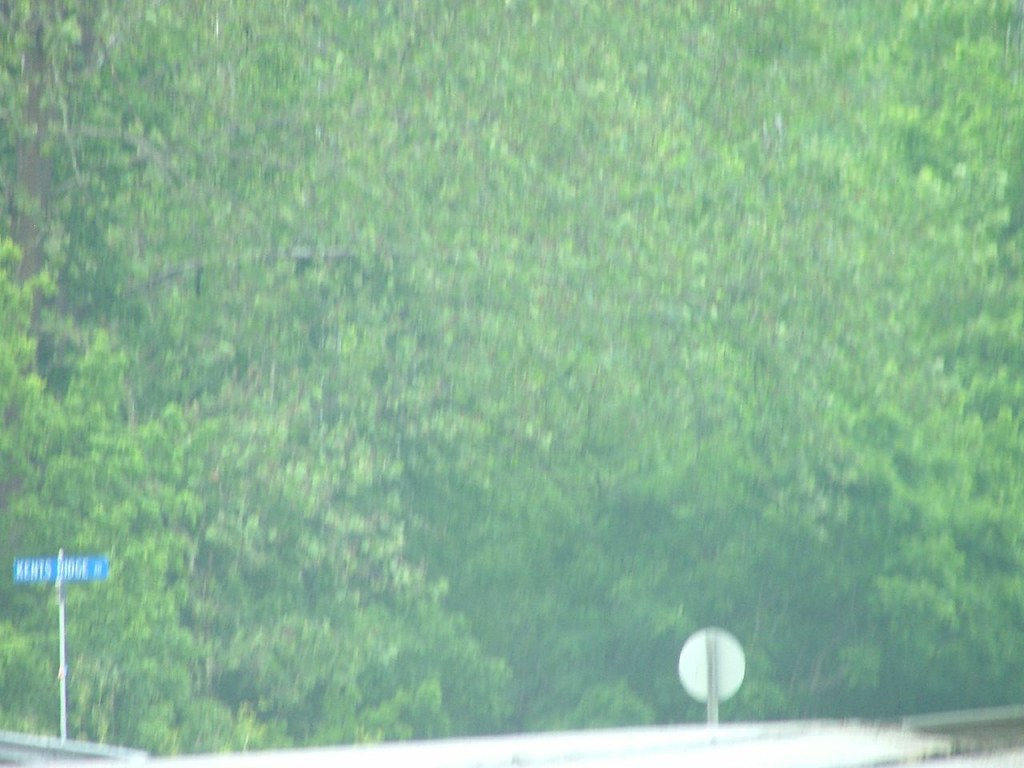This blurry and overexposed color photograph appears to have been taken from inside a moving car, capturing the side of a road on a bright, sunny day. Dominating the image is a flat, expansive area filled with trees and dense foliage, with leaves prominently in view. At the very bottom, shadowing creates a slight contrast, hinting at the presence of a guardrail, which is partially visible. Positioned slightly to the right of the center at the bottom of the image is the backside of a round street sign mounted on a metal pole. To the left at the bottom, there is a blue street sign that reads "Kent's Ridge Road." Despite its low quality, the photograph offers a fleeting glimpse of a roadside landscape.